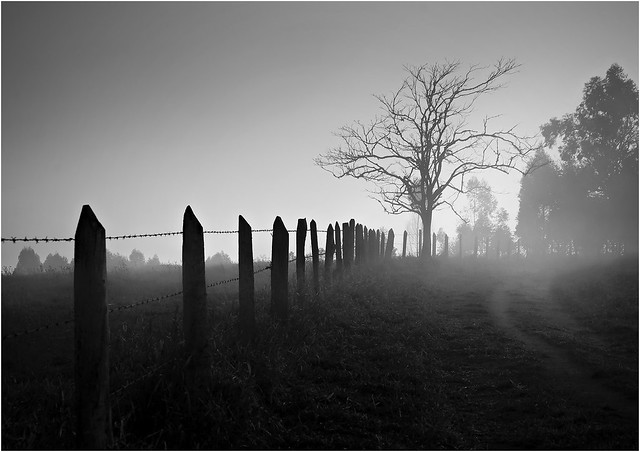The image is a black-and-white landscape photograph capturing an outdoor scene during either sunrise or sunset. The sky transitions from dark to light, creating a gradient that highlights the horizon about halfway down the composition. Dominating the center-right is a striking dead tree with multiple branches, silhouetted against the subtly lightening sky. Flanking this tree are pines to the right and additional trees to the left, all reduced to gray shapes in the monochrome palette. A white mist drifts across the horizon and towards the central point from the top right, adding a ghostly ambiance. 

In the foreground, a fence extends from the bottom-left corner towards the center, lined with at least three strands of barbed wire, then curves to the right, disappearing into the woods at the top right. Also notable is a dirt trail that winds in from the right side, gently curving leftward before disappearing into the trees. The photograph’s representational realism and meticulous grayscale detail enhance the haunting tranquility of the rural landscape.